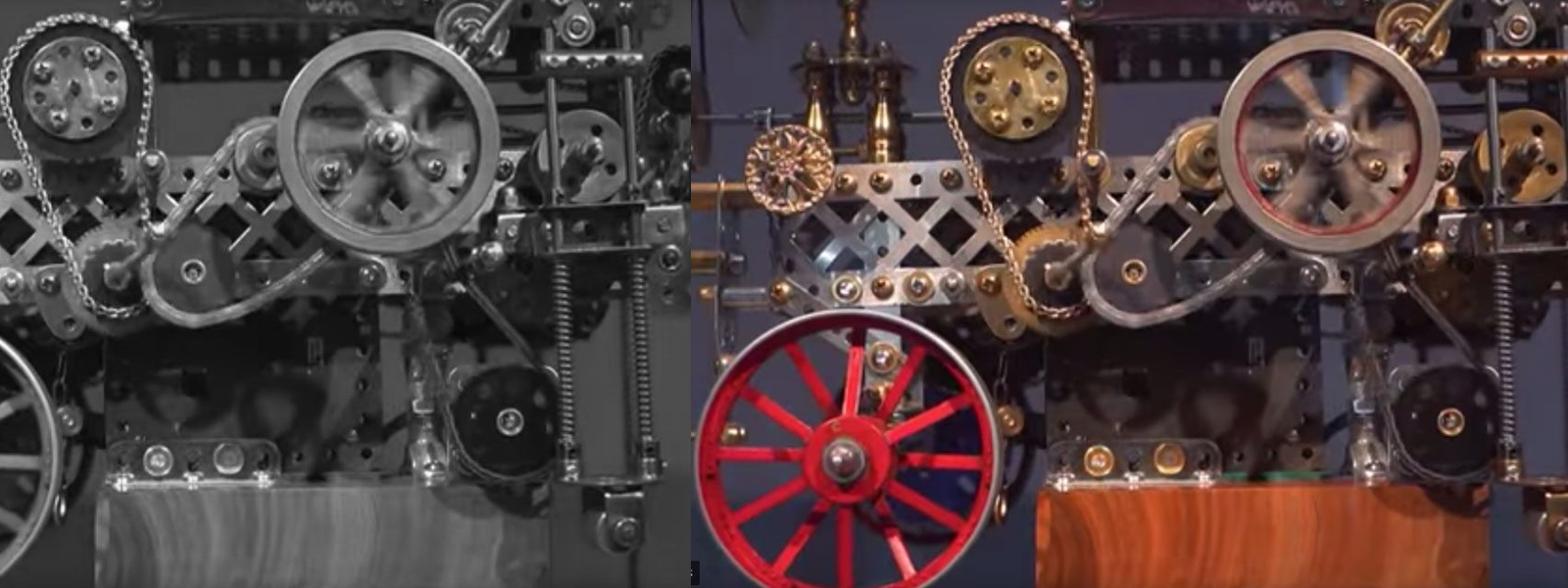This image showcases a vertically elongated picture consisting of two nearly identical photographs placed side by side. The photograph on the left is in black and white, while the one on the right is in color. Both images depict an intricate and busy mechanical machine, featuring numerous wheels, gears, chains, and spokes of varying sizes and colors. The machine's components are primarily in rose gold, shiny silver, and gold hues. Notably, there is a red wheel on the bottom left of the colored portion, trimmed in silver. The machine appears to be more artistic in nature rather than functional. A smaller wooden table or box sits beneath the machine, which further adds to the complexity and intentional design of the setup. The background wall is gray, providing a neutral backdrop that highlights the vivid colors and metallic details of the machine.